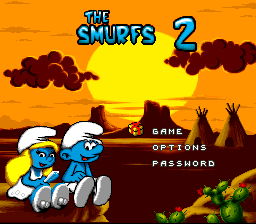The screenshot captures a scene from the video game "The Smurfs 2," indicated by the title in blue at the top of the image. The scene depicts a vivid desert sunset with an orange sky dominated by a large, bright yellow sun partially obscured by brown clouds. The background showcases rock formations resembling badlands or mesas and two teepees, further emphasizing the desert setting. In the lower left corner, two blue Smurfs are seated on a bluff. The Smurf on the left has long blonde hair, wearing a white hat, white shirt, and white shoes, while the one on the right wears a white hat and white pants, but no shirt. There is also a dead branch and a cactus with red blooms in the lower right corner. A menu is displayed in the middle right of the image with options "Game," "Options," and "Password" printed in white.